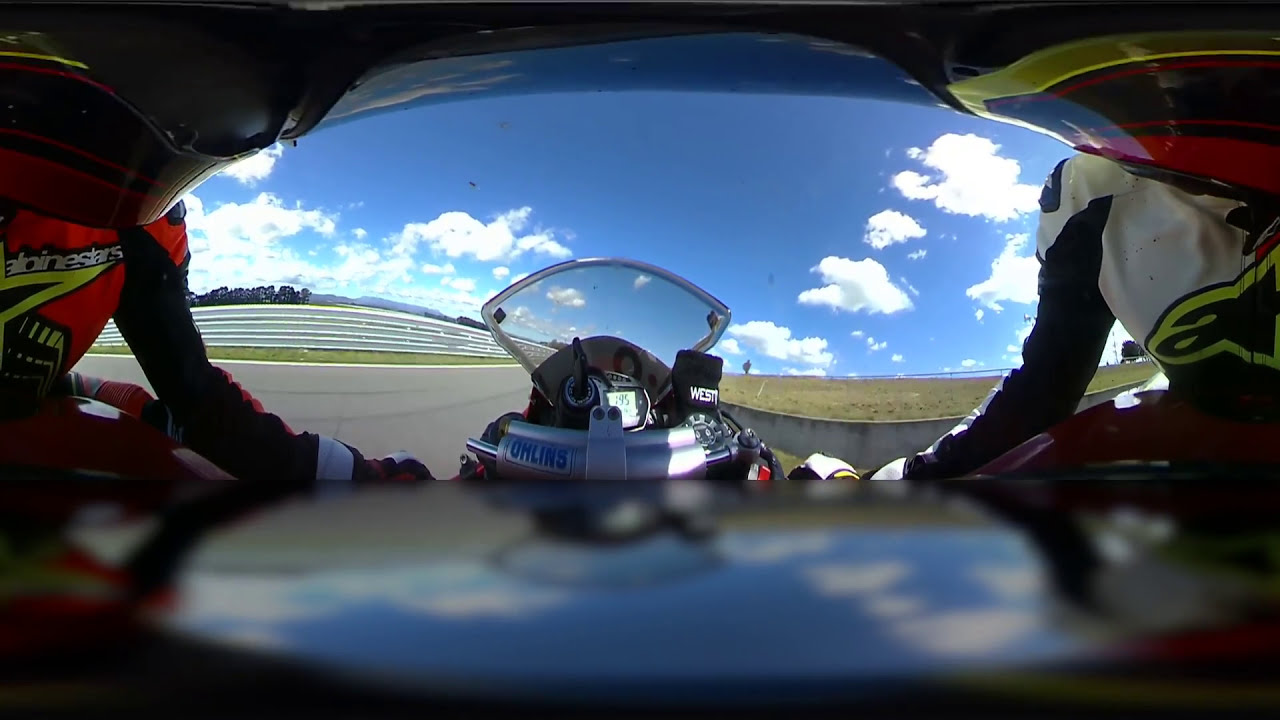In this detailed panoramic image, we are looking from the front of a sleek, low-riding, single-person vehicle, possibly a motorcycle. The vehicle's dashboard features a prominently displayed gauge reading 195, flanked on the right by a glove bearing the word "West" with a small circular detail below it. Below the speed gauge are two white tubes, the bottom one inscribed with "OHLINS." The surface of the vehicle is just visible below this complex setup.

To the left and right of the vehicle, we see two figures, appearing to be either engineers or fellow riders, suggesting a setting filled with professionals. The person on the left wears a black helmet and an orange shirt emblazoned with "ALPINESTARS." The person on the right is clad in a red and yellow shirt, layered with a white and yellow shirt that has an "A" on it. 

The background extends into a landscape featuring blue skies with bright white clouds, indicating a sunny day. On the far right, a concrete wall is visible, while to the left, a metal barricade lines the road, leading the eye towards distant trees and the expansive sky. The riders' heavy jackets add to the impression of speed and movement in this dynamic scene.